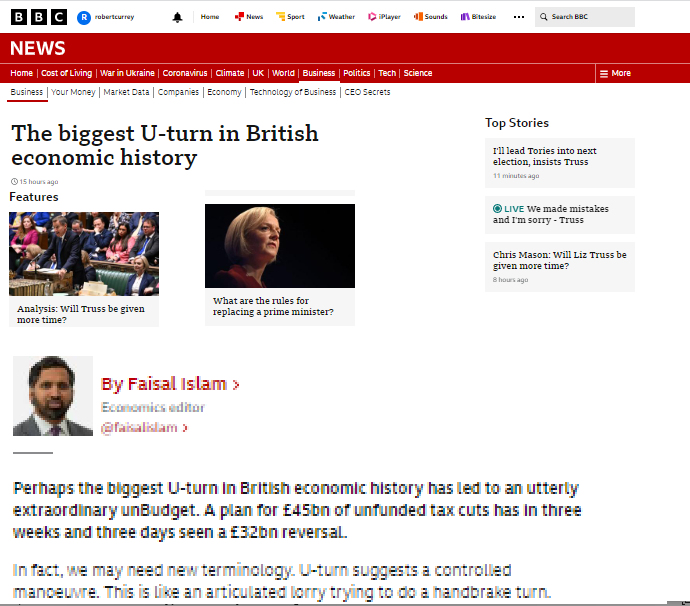The image is a screenshot of the BBC News website, captured from someone's computer. The screenshot displays a slightly rectangular layout rather than a perfect square. At the top, it prominently features the BBC logo set against a white bar that includes notifications and various sections of the website. Below the white bar is a red navigation bar that categorizes content with labels such as "News," "Home," "Cost of Living," "War in Ukraine," "Coronavirus," "Climate," "UK," "World," "Business," "Politics," "Tech," and "Science," all in small white text.

Centrally positioned within the image is a larger headline in black text stating: "The biggest U-turn in British economic history." This headline is set against a clean, white background. To the right, a section labeled "Top Stories" features additional headlines: "I'll lead Tories into the next election, insists Truss (Live)," "We made mistakes, I'm sorry, says Truss," and "Chris Mason: Will Liz Truss be given more time?"

Beneath the main headline, there is a photo of Liz Truss, followed by an image of a man speaking in Parliament, and another blurry photo depicting what appears to be an Indian man. In red text, the caption identifies the article's author as "By Faisal Islam, Economics Editor." The remaining part of the screenshot includes some of the article's text, providing further context to the headline.